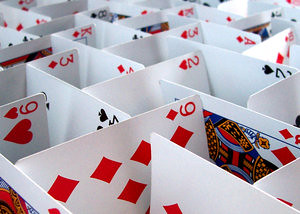A meticulously arranged series of playing cards is showcased from a slightly downward angled perspective, creating an intricate visual resembling a maze or labyrinth. The cards are meticulously staggered, forming a striking pattern reminiscent of winding pathways and blocked passages, although clearly not intended as an actual maze. 

Each card stands either vertically or horizontally, with a vertical card typically meeting a horizontal card at its edge, continuing this interlocking pattern throughout the arrangement. This rhythmic repetition of vertical and horizontal cards generates an elaborate and visually engaging layout.

At the forefront of the display, several cards are distinctly visible: the nine of hearts, nine of diamonds, queen of diamonds, two of hearts, three of diamonds, four of diamonds, two of spades, four of spades, ace of diamonds, ten of diamonds, king of diamonds, king of hearts, and eight of spades. The vivid contrast between the red hearts and diamonds and the black spades and clubs further emphasizes the complexity and aesthetic appeal of the card configuration, making it a captivating focal point.